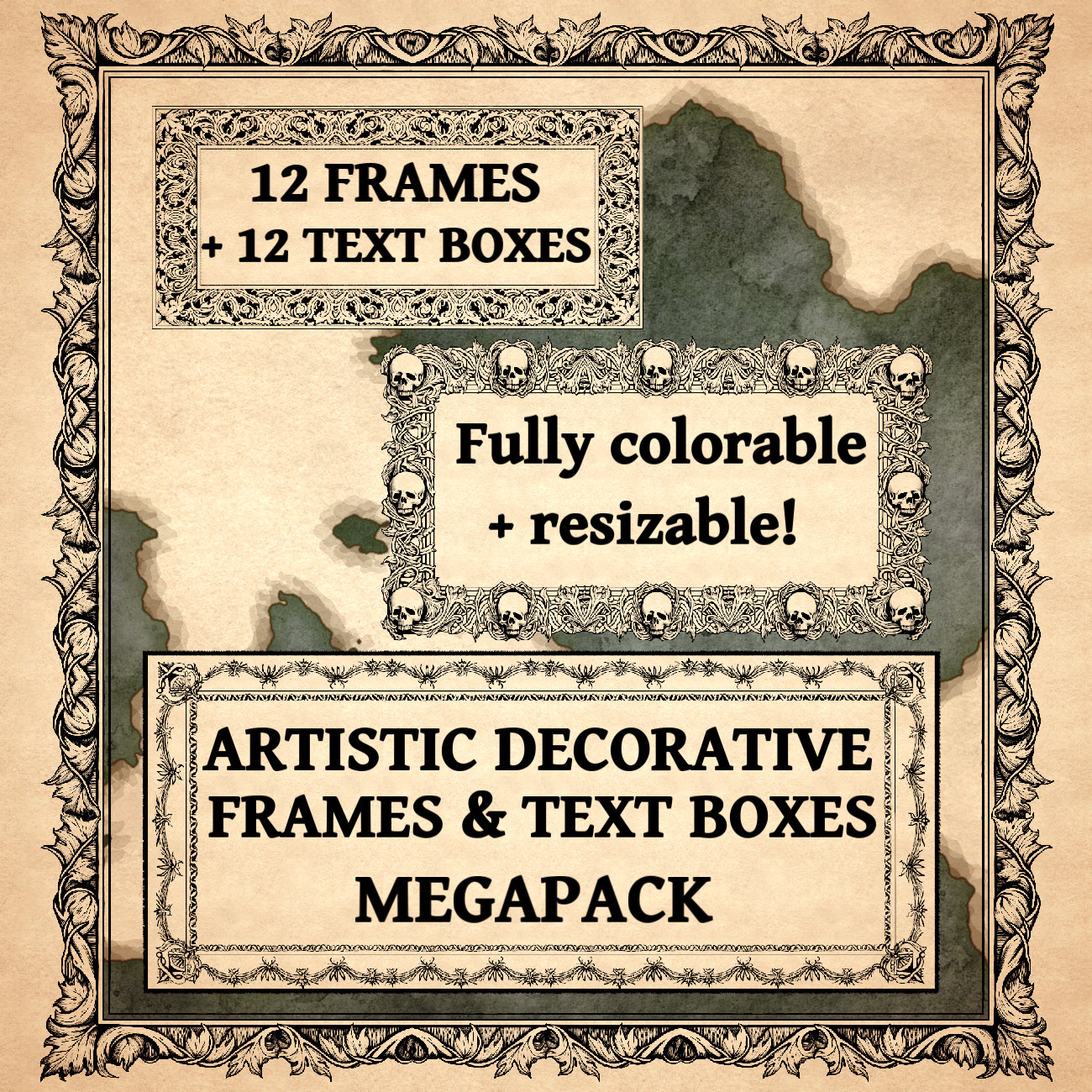The image resembles an old-fashioned advertisement with a parchment beige background. It is a vertical rectangle, inside which another smaller black rectangle is framed by intricate black scrolling and leaf designs. This ornate filigree continues around three smaller horizontal rectangles within the black frame. The top rectangle reads "12 frames plus 12 text boxes" and is surrounded by a similar filigree design. The middle rectangle, bordered by evenly spaced skulls and bones, announces, "Fully colorable and resizable!" The bottom rectangle, encircled by a vine-like pattern, promotes the "Artistic Decorative Frames and Text Boxes Mega Pack." The overall image conveys a vintage aesthetic with detailed decorative elements and text boxes, ideal for a promotional poster.